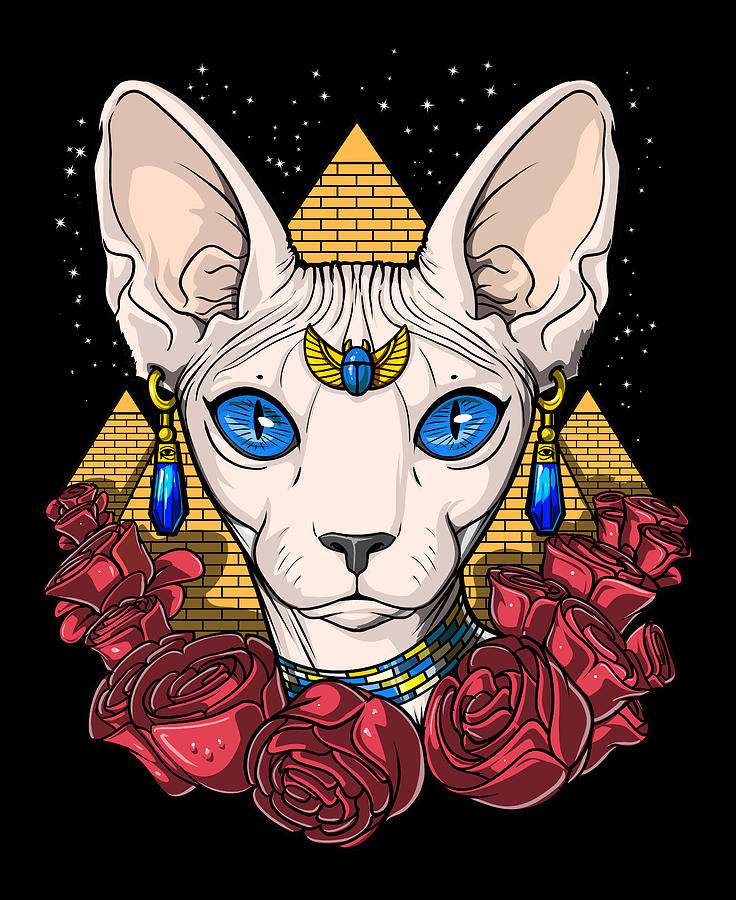This vibrant computer-animated image features a stylized, Egyptian-themed depiction of a hairless cat with a cartoonish design. At the center, the tan-colored cat's head is prominently displayed, revealing its distinct large ears, wrinkled skin, and mesmerizing, wide-open blue eyes. Adorning the cat are sophisticated accessories: golden earrings with blue pendants, a colorful beaded necklace of blue, gold, and white bands, and an intricate blue and gold scarab beetle positioned on its forehead. Encircling the feline are lush red roses, adding a startling contrast to the image. Behind the cat, golden pyramids, rendered in a stylized, non-realistic manner, rise against a stark black sky sprinkled with several twinkling stars, further enhancing the mystical and alluring Egyptian aesthetic of the artwork.